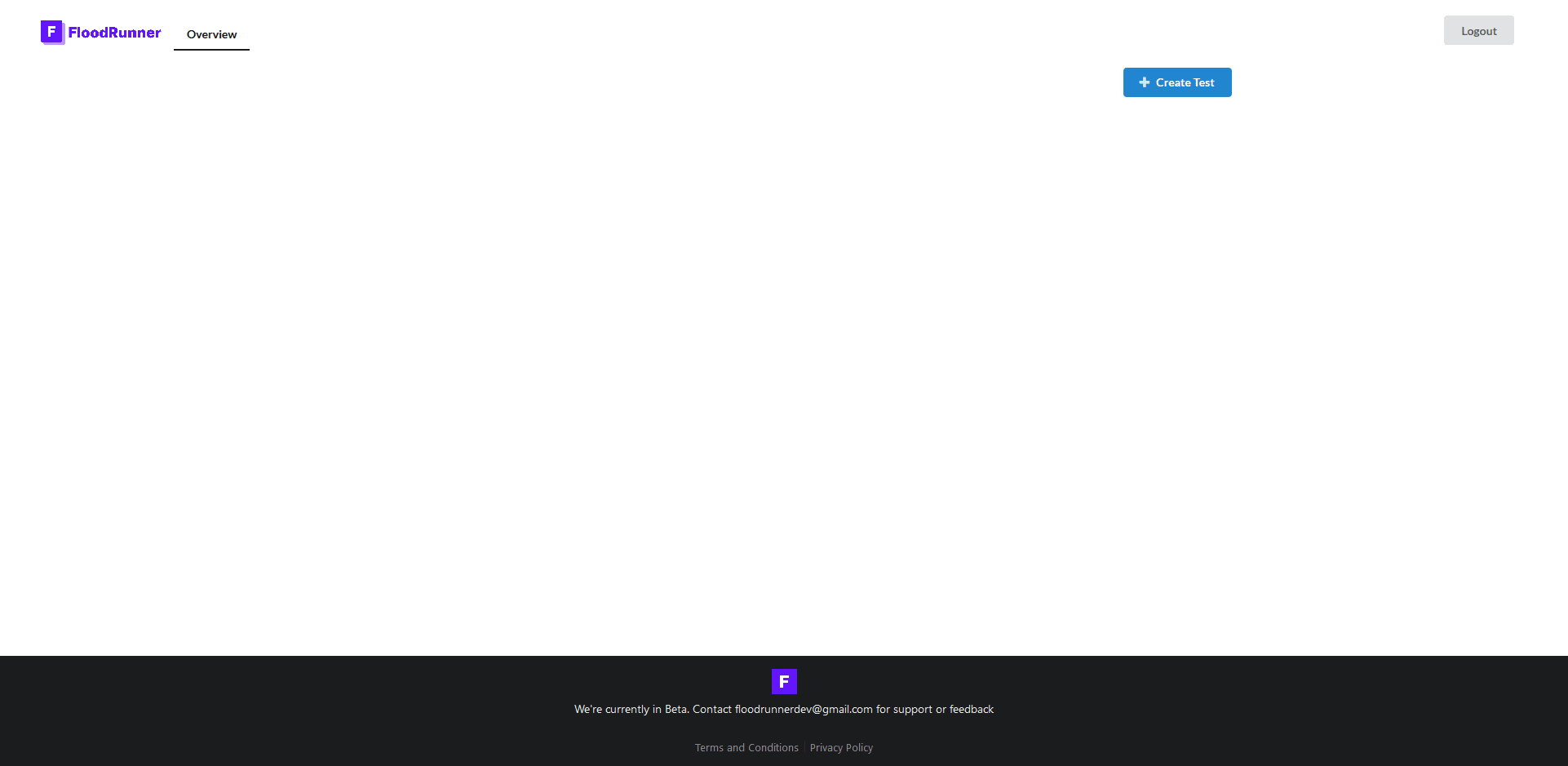The image depicts a screenshot set against a white background featuring an interface with various elements. In the upper left corner, there's a logo consisting of a white "F" inside a purple box, accompanied by the text "Flood Runner" in purple. Adjacent to the logo in gray text is the word "Overview," underlined by a gray line. To the right of "Overview," there's a blue rectangular action button with a white plus sign icon and the text "Create Test." In the upper right corner, there's another action button for logging out, presented in light gray with dark gray text. At the bottom of the screen, a black footer spans the width of the image, displaying a blue square with a white "F" icon. Below the icon, in small white text, it reads: "We're currently in beta. Contact floodrunnerdev@gmail.com for support or feedback."